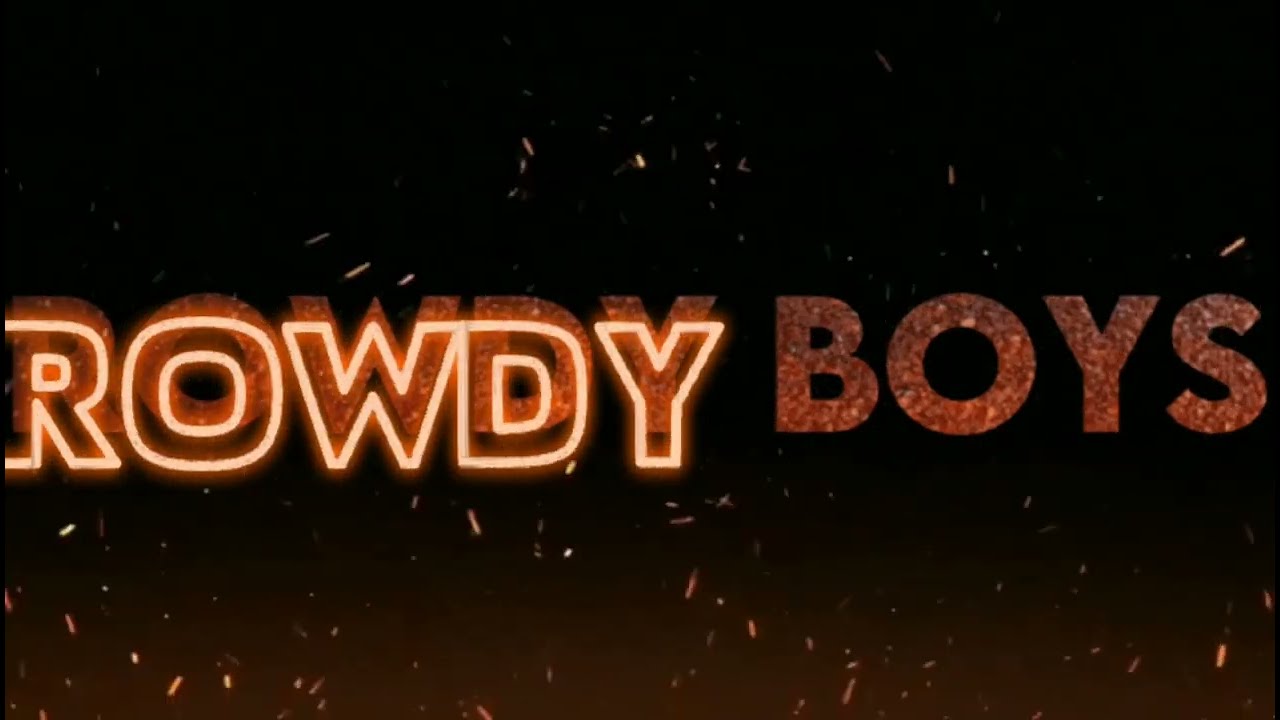The poster predominantly features a black background, illuminated from the bottom with fiery hues suggesting embers or sparks from an unseen bonfire. These flickers of reddish-orange light scatter throughout the image, giving it a dynamic and intense atmosphere. Central to the design is the text "ROWDY BOYS" in capital letters. The word "ROWDY" appears in a striking 3D effect, outlined in white and glowing with a neon-like orange light, making it stand out prominently against the darker backdrop. Below "ROWDY," the word "BOYS" appears, rendered charred or weathered, lacking the 3D effect but still vivid with burnt orange and red elements. The overall composition suggests a logo or banner, possibly for a TV show, band, or organization, characterized by its bold and dramatic presentation.